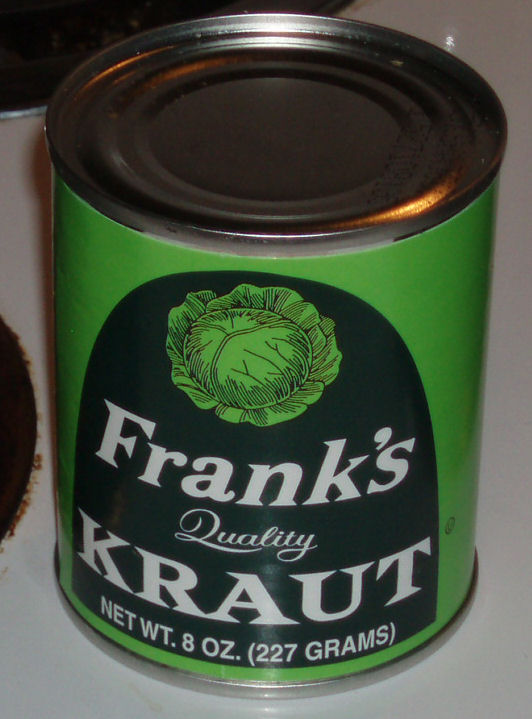The color photo showcases an unopened can of Frank's Quality Kraut, prominently featuring a green label. The label includes a darker green shade toward the top with an image that appears to be green cabbage. The text on the label reads "Frank's" in large white letters, "Quality" in smaller white letters—though the Q might look like a D to some viewers—and "Kraut" in large white letters below. The can indicates a net weight of 8 ounces (227 grams). The silver, unopened top of the can suggests it requires a can opener for access. The can rests on a white surface, likely a table or counter, with a partially visible, possibly dirty black burner or stove to the left and an indistinguishable brown object. The top of the can also has some small, unreadable text.